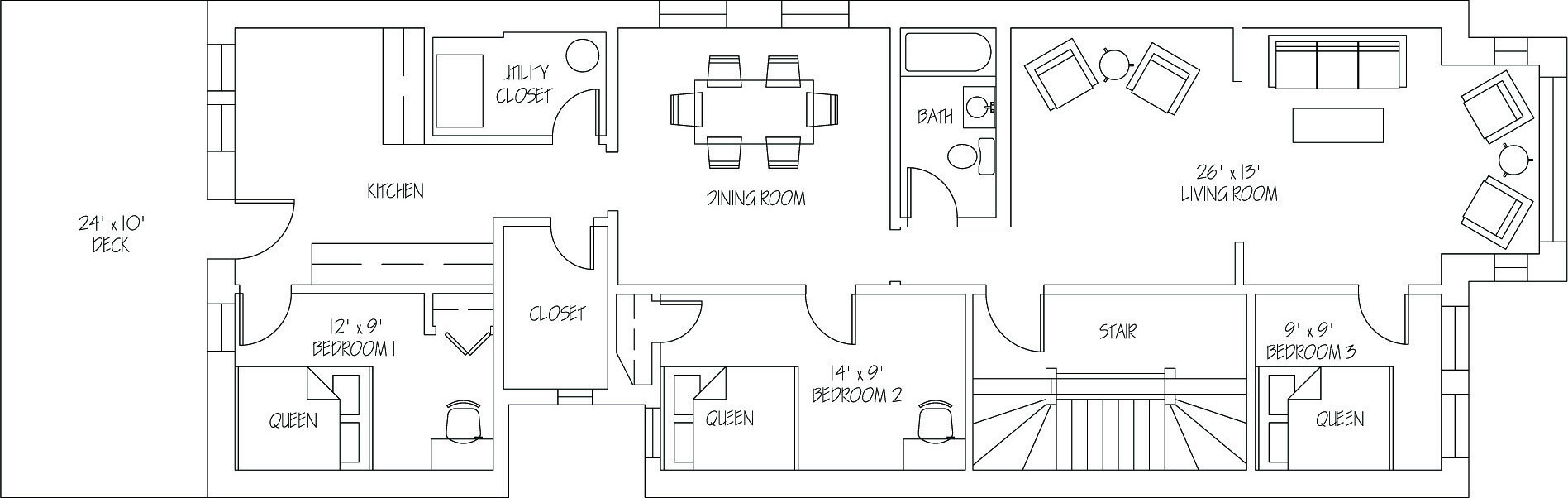The image depicts a detailed floor plan of a ranch house with a white background and black lines. The plan includes a 24-foot by 10-foot deck located on the left side, which seems to be the main entrance. A door to the right of the deck leads directly into a kitchen equipped with counters. Adjacent to the kitchen on the right is the first bedroom, measuring 12 feet by 9 feet, complete with a queen bed and a small closet. 

Returning to the kitchen and proceeding down the hall on the left, there is a utility closet possibly containing a water heater and washer/dryer hookups. To the right of the hall is a deeper, walk-in closet. Further down is the dining room that features a table with six chairs. From the dining room, the second bedroom can be accessed, measuring 14 feet by 9 feet and also accommodating a queen bed.

Continuing through the hallway, directly adjacent to the dining room, is a bathroom fully outfitted with a tub, sink, and toilet. Past this point, a doorway and stairs likely lead to a basement. Further along is the spacious living room, measuring 26 feet by 13 feet. The living room is divided into sections: one with chairs, another with a couch and coffee table, and a small adjoining area with two additional chairs. Lastly, the third bedroom is accessible from the living room, measuring 9 feet by 9 feet and fitting a queen-size bed.